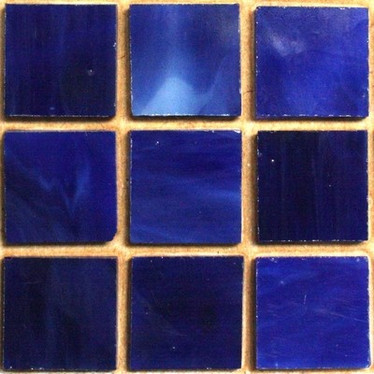The image features nine distinct blue tiles arranged in a three by three grid against a beige or tan background, reminiscent of a checkerboard or one side of a Rubik's Cube. Each tile showcases a different shade of blue, ranging from bright cerulean to dark indigo and marine blue. Some tiles are accented with white blobs or striations, adding texture and variation. The tiles, possibly made of lucite or a similar material, are separated by thin grout lines, enhancing the individuality of each square despite their cohesive arrangement. The entire composition evokes a sense of unified diversity through the varying hues and patterns within the blue color family.